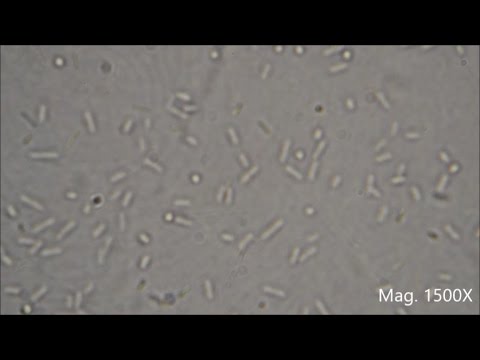The image is a highly magnified, blurry slide viewed under a microscope at 1,500 times magnification, as indicated by the text "MAG 1500X" on the image. The slide displays what appear to be small, cylindrical objects resembling grains of rice, which could be tubule-shaped bacteria or molecules. In addition to these, there are also smaller, spherical shapes suggesting a mix of different types of bacteria, all set against a splotchy dark gray background. The image has a black bar running along the top and bottom edges, giving it a scaled, almost low-resolution video frame appearance. The objects and background are depicted in varying shades of gray and white, making it hard to identify the specifics without further context. Overall, the image captures a chaotic scatter of these microscopic entities, numbering approximately 120 across the entire slide.